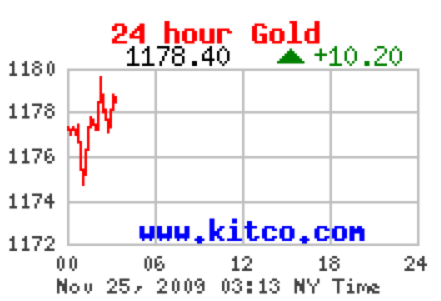The image is a detailed graphic charting the price of gold over a 24-hour period. At the top of the graphic, prominently displayed in red text, is the title "24-Hour Gold." Below this title, the current price of gold is shown along with an increase of $10.20, depicted with a green arrow for emphasis, indicating a positive trend. The price displayed is $1,178.40. 

The vertical axis, labeled in black or gray, ranges from $1,172 to $1,180, marked at intervals of 2. The horizontal axis at the bottom of the graph displays time in hours, from 0 to 24, marked in 6-hour increments. The line graph indicating price changes shows a jagged, fluctuating red line which trends upwards overall. Initially steady, the price graph shows a drop before rising consistently between hours 00 and 06.

Additionally, at the bottom of the chart, the date "November 25, 2009," along with the specific time "3:13 New York time," is indicated, providing a clear timestamp for the data presented. The graph also includes the website address www.kitco.com.